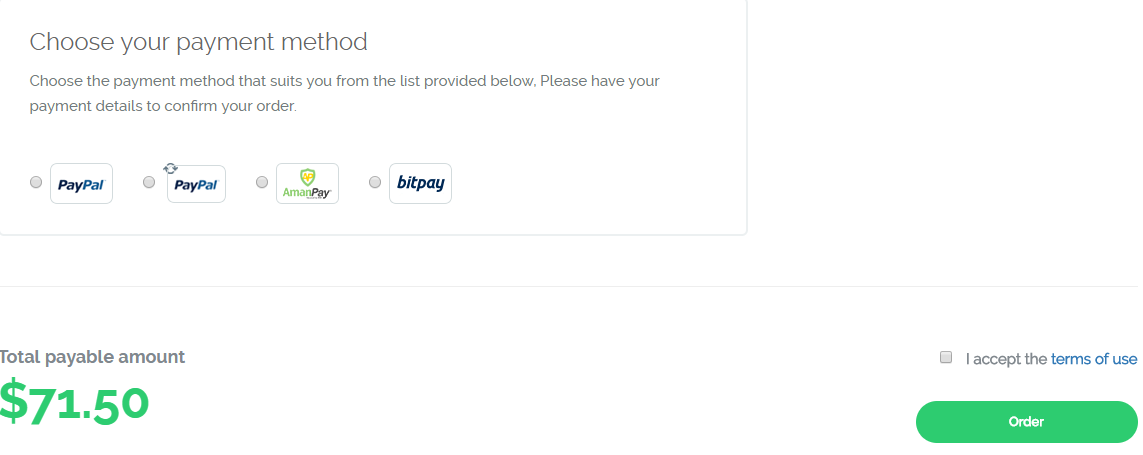The image features a clean, white background. At the top, there's a blue-outlined box that contains text: "Choose your payment method. Choose the payment method that suits you from the list provided below. Please have your payment details to confirm your order." Below, there are selection circles for different payment options including PayPal (with an additional slightly varied PayPal option), Amazon Pay, and BitPay. Each payment option is preceded by a circular checkbox for selection.

In the upper left corner of the image, there is a small diamond shape. Farther down, a prominent blue line separates the payment options from the total payable amount, which is displayed in green text as "$71.50". 

On the right side, there's a small blue box with a checkbox labeled "I accept the terms of use". Below this is a green button labeled "Order". 

The layout clearly presents the payment process with the options prominently displayed for ease of selection, and provides a clear call to action to complete the order.